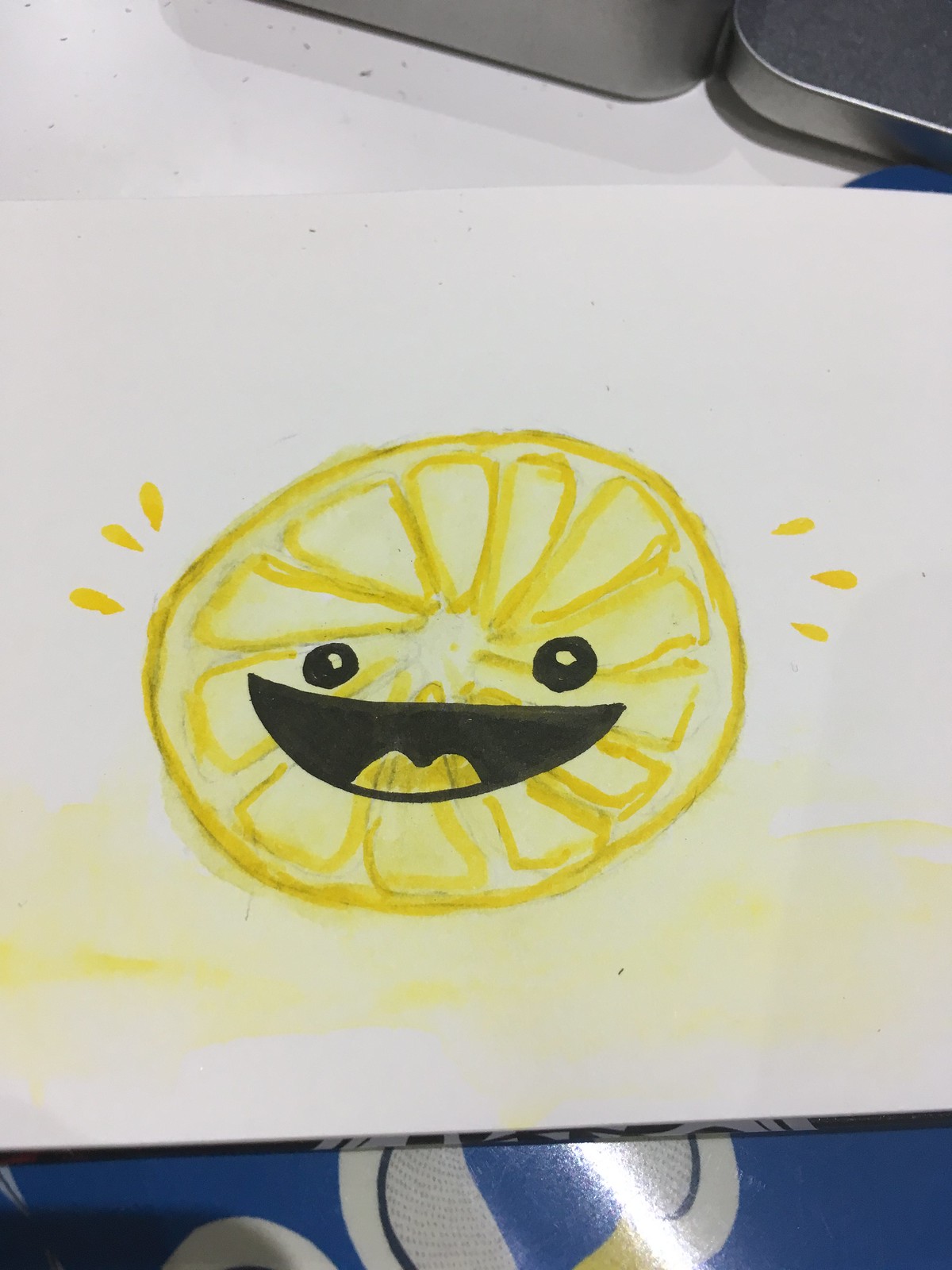This image features a playful and artistic rendition of a lemon, skillfully drawn yet retaining a simple charm. Created likely with a yellow marker, the lemon is depicted sliced in half, revealing a whimsical face. The face, illustrated in black, includes open eyes and a smiling mouth with a visible tongue. To enhance its lively appearance, three droplets are drawn on each side of the lemon, suggesting freshness or a burst of juice. The lemon is placed on a shaded yellow backdrop, adding a subtle depth and anchoring the character in the scene.